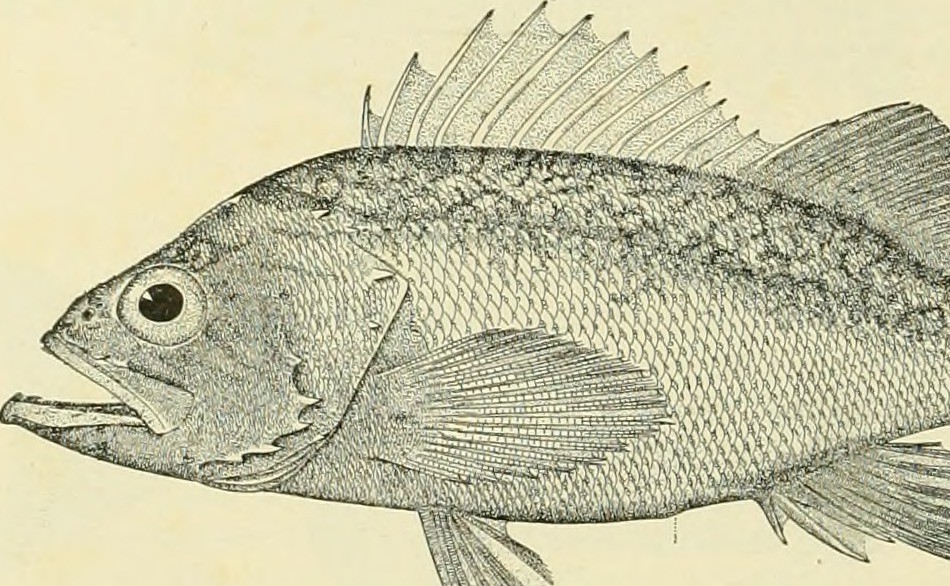This hand-drawn image of a large fish, facing left, dominates the scene with its impressive black ink detailing against a yellow, grayish-teal, or beige background. The fish is meticulously illustrated, showcasing a variety of textured scales that differ from the top to the underbelly. Its wide eye, a striking dark circle, is positioned just above the open mouth, enhancing its expressive appearance. A sharp, pointed fin runs along the top from about one-third to two-thirds of the body, followed by a smoother, darker fin toward the back. Centrally located is a prominent swimming fin, balanced by a smaller fin below it, and farther back on the underside is another large, pointed fin. The composition is highly detailed, capturing the intricacies of the fish's gills, scales, and other minute features, all stylized with a sense of hand-drawn artistry, making the image stand out without the need for any accompanying text.